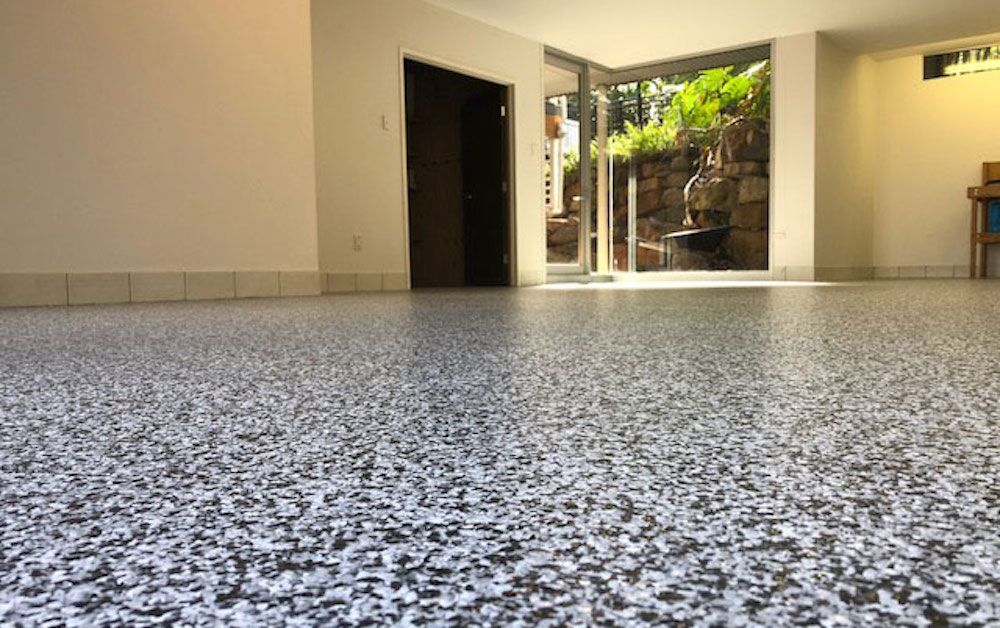The photograph taken during the daytime shows the interior of a building with a focus on the lower half of the scene. The floor features a marbled or rock-like pattern in shades of white, black, and gray. The top half of the image reveals a beige or creamy white wall with a white tiled trim at the bottom. Slightly to the left is an elevator door, darkened and centered within the frame, next to which is a light switch and plug. To the right of the elevator is an open door leading to a dimly lit room. Further to the right is a floor-to-ceiling window revealing an outdoor area with a rock wall and bright lime green plants. The far right of the image shows an alcove with a wooden chair featuring a bluish backrest for support, positioned below another window that brings in natural light.